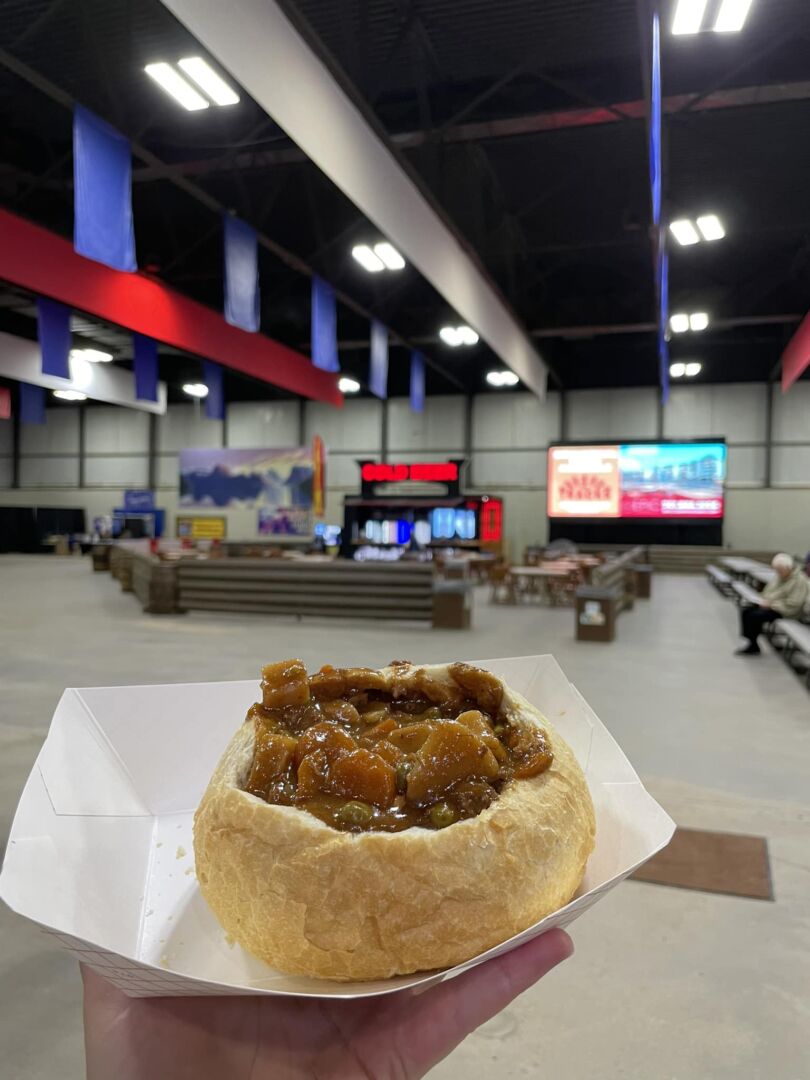A man is captured during his lunch break, holding up a savory bread bowl filled with soup or chili in his left hand. The bread bowl is nestled in a white rectangular disposable paper basket. The background reveals a large, sparsely populated open space with high, dark ceilings and gray walls, suggesting a multi-purpose venue such as a trade show or convention center. The floor is smooth concrete. A large LED screen or projector displays content, presumably for guests dining or attending an event. Various tables and benches are scattered around with very few people present, including one person on the right engrossed in a paper or informational sheet. Blue flags hang from the ceiling, and there are stations that might be for refreshments like cold beer.